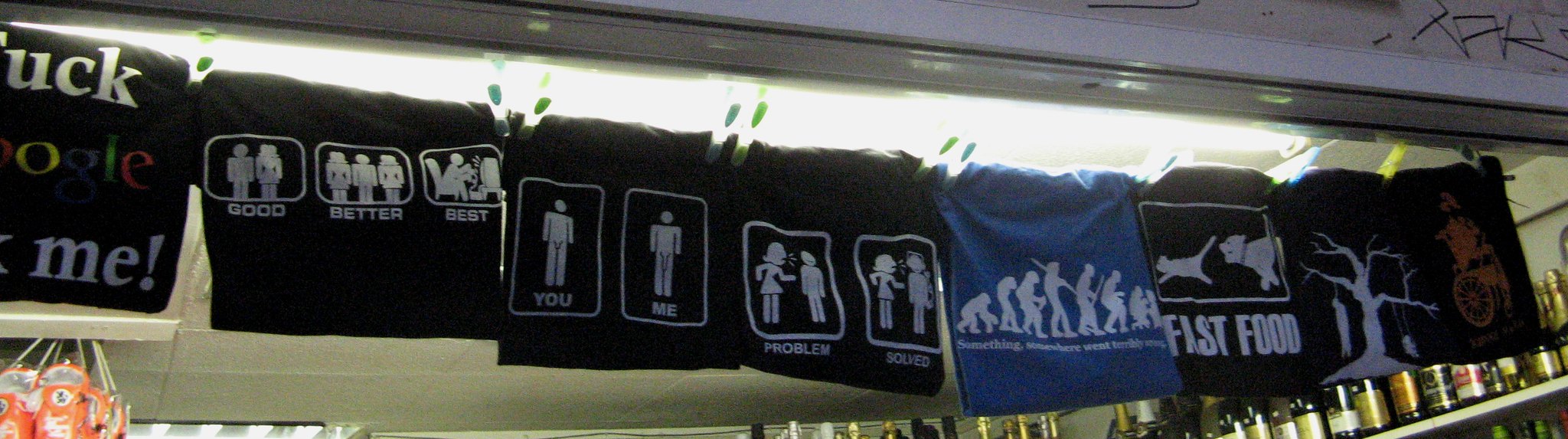The photo captures the interior of a quirky convenience store, specifically focusing on the ceiling, where an array of novelty t-shirts are displayed in place of typical signage. The majority of these t-shirts are black, each printed with a unique and often humorous image or phrase. Among them, one shirt features the phrase "fuck Google me," while another illustrates three scenarios labeled "Good," "Better," and "Best" with stick figures: a couple, a trio including two women, and a woman riding a man in front of a TV. Another shirt shows the evolution of man culminating in a gamer at a computer. Other designs include a stick figure comic with the phrases "You" and "Me," a problem-solving sequence with a man using headphones to block out a yelling woman, a "Fast Food" graphic of a dog chasing a cat, an ominous tree with two people hanging from it, and a steampunk Dalek. In the background, shelves stocked with alcohol bottles are visible, adding to the eclectic mix of the store's offerings.